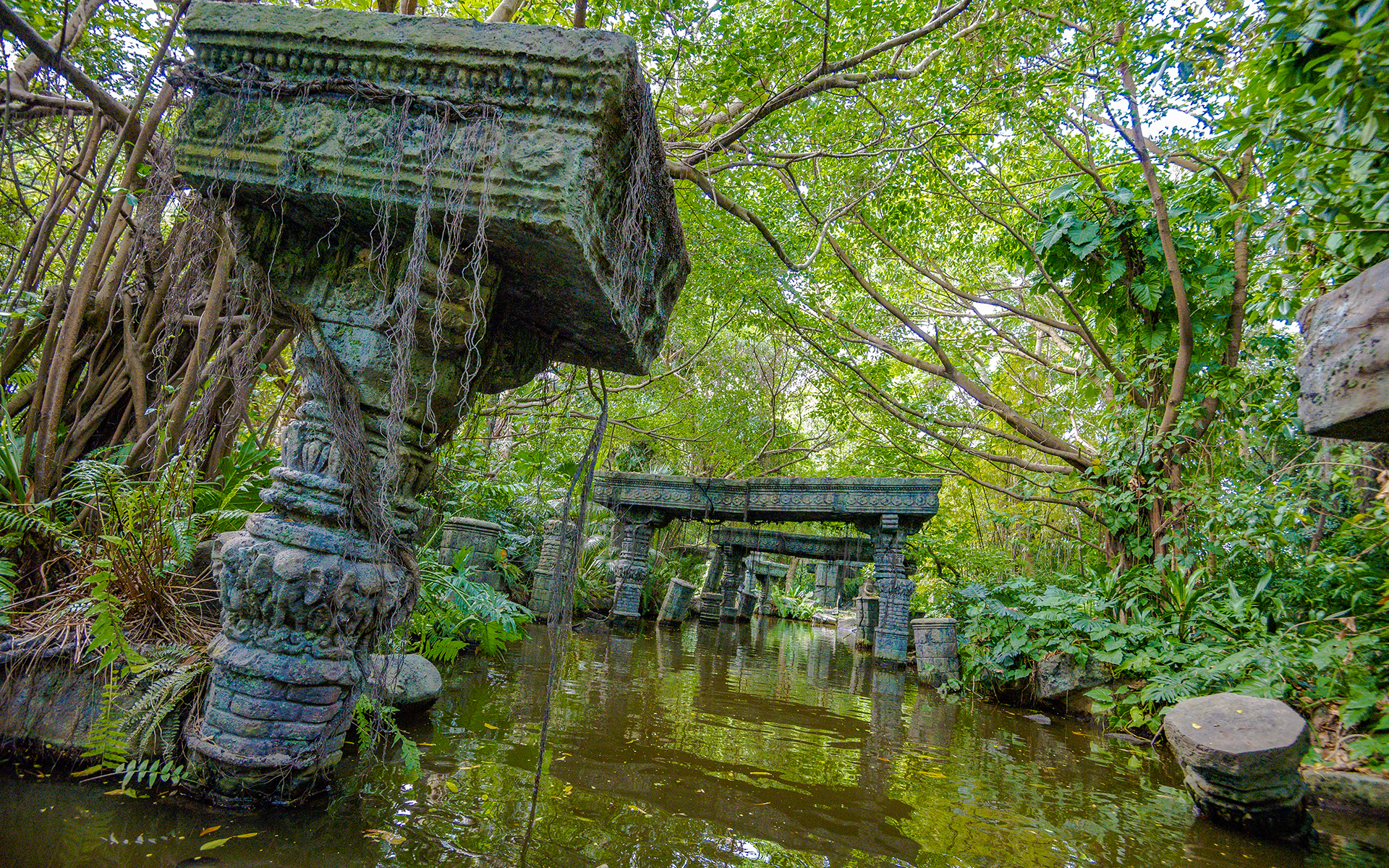The photograph captures a serene water canal meandering through a lush, forested landscape reminiscent of a rainforest. The canal's still, yellowish-green water is dotted with floating dead leaves, adding a touch of natural decay. Along the banks stand a series of ancient, dramatic stone pillars, some with ornate features, hinting at a bygone era of architectural grandeur. These pillars, weathered by time, appear to be remnants of old bridges, now broken and overtaken by nature. The pillars are varied, with some topped by square platforms and others draped in dead vines. Interspersed among these columns are occasional arches, further emphasizing the sense of historical ruin. Surrounding this canal, a dense array of greenery—including towering trees, ferns, vines, and shrubs—envelops the scene. Pockets of bright sky peek through the thick canopy, illuminating the tranquil yet eerie ambiance of the forgotten, flooded structures.